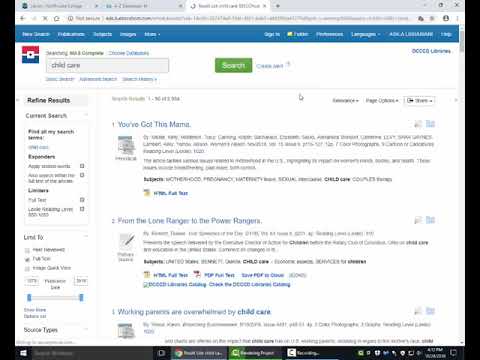The image features a website webpage. At the top of the page is a green search bar with the word "childcare" typed into it. The company's logo is displayed prominently and consists of a rectangular box divided into three sections: a red top, a blue bottom, and a white box in the middle. 

The browser and main search bar contain unreadable text, but nearby is a section labeled "Rating Results" and "Customer Search." There's also a link or button that says "Find" followed by unreadable text.

In the main body of the webpage, several entries are visible:

1. The first entry briefly mentions "You've got a thin Marma" and includes a picture alongside a description, though the text is too small to read.
   
2. The second entry is titled "From the Lone Ranger into the Power Rangers" and has its own accompanying image and description, which are similarly unreadable due to small font size.

3. The third entry is titled "Working Partners are Overwhelmed by Childcare" and features an image and a description in gray text, which again is too small to be legible.

In the upper right corner of the page, there is additional text mentioning "libraries," but the complete context is not discernible.